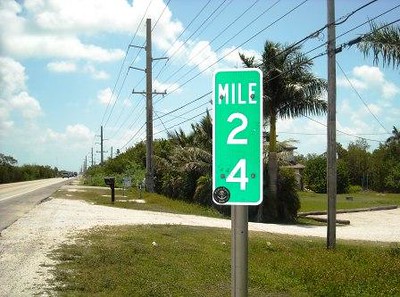The image prominently features a road sign reading "Mile 24," which is arranged vertically with "Mile" at the top followed by "2" and "4." This sign stands in a lush, tropical environment, as evidenced by the numerous palm trees and dense greenery that frame the scene. To the right of the sign, tall palm trees and other bushy plants thrive, creating a vibrant swath of green. Extending from the right to the left side of the image, a series of telephone poles cuts across the landscape, diminishing into the distance. The road itself is partially visible on the left side, with a few cars traveling along it. Additionally, a stony path diverges from the road, leading off to the right of the sign, adding an element of intrigue to the setting.